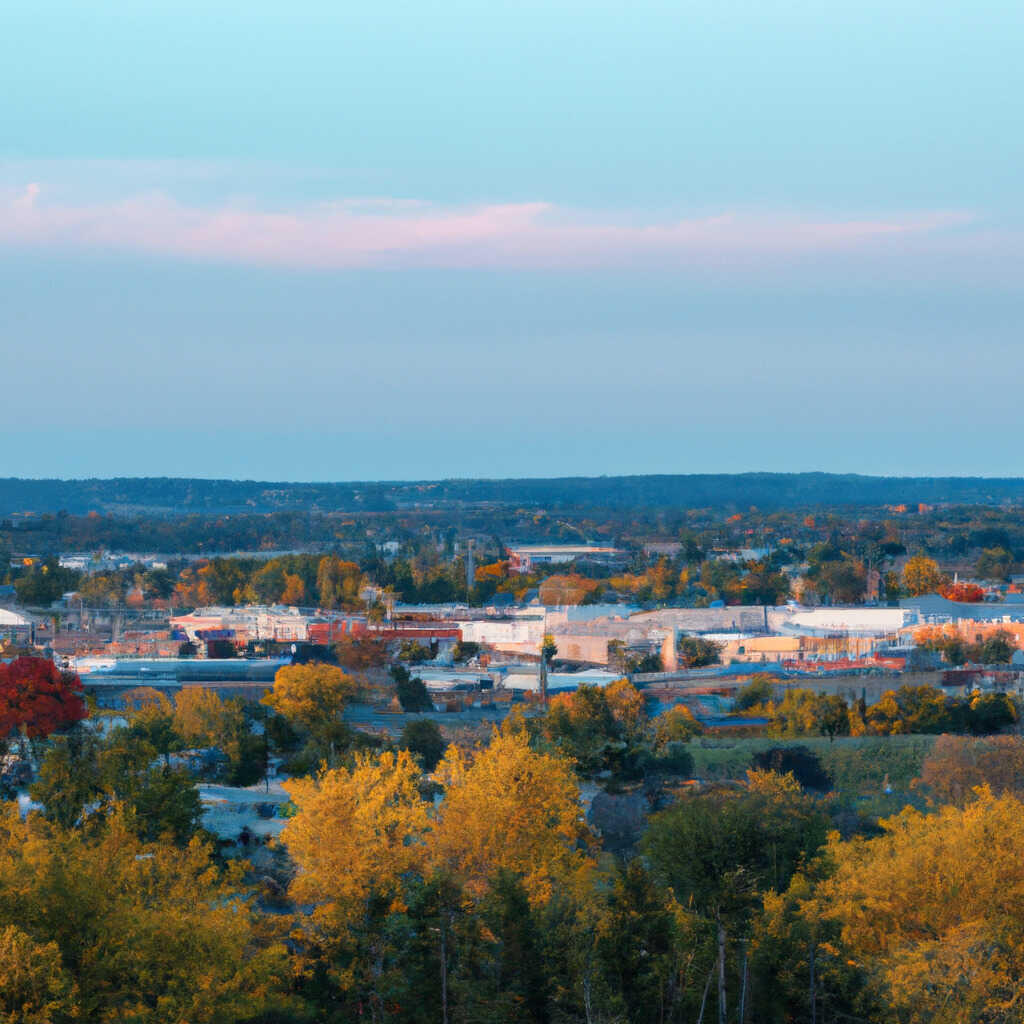The image captures an elevated view, likely taken from a hill, overlooking a small town or village nestled at the bottom of the scene. Scattered among the buildings, which feature white and gray roofs, are numerous trees displaying a vibrant mix of fall colors—bright yellows, oranges, with a strikingly red tree on the left side, interspersed with some still-green foliage. The photograph appears to be taken during late afternoon with a light blue sky overhead, contributing to the tranquil ambiance. The sky is filled with varying cloud formations including light gray haze and whiter clouds slicing horizontally across the scene. In the mid-ground, amidst the autumnal trees, some larger buildings stand out, possibly indicating facilities like schools or factories. The overall composition beautifully blends the community infrastructure with the surrounding nature, capturing the seasonal transition in a serene landscape.